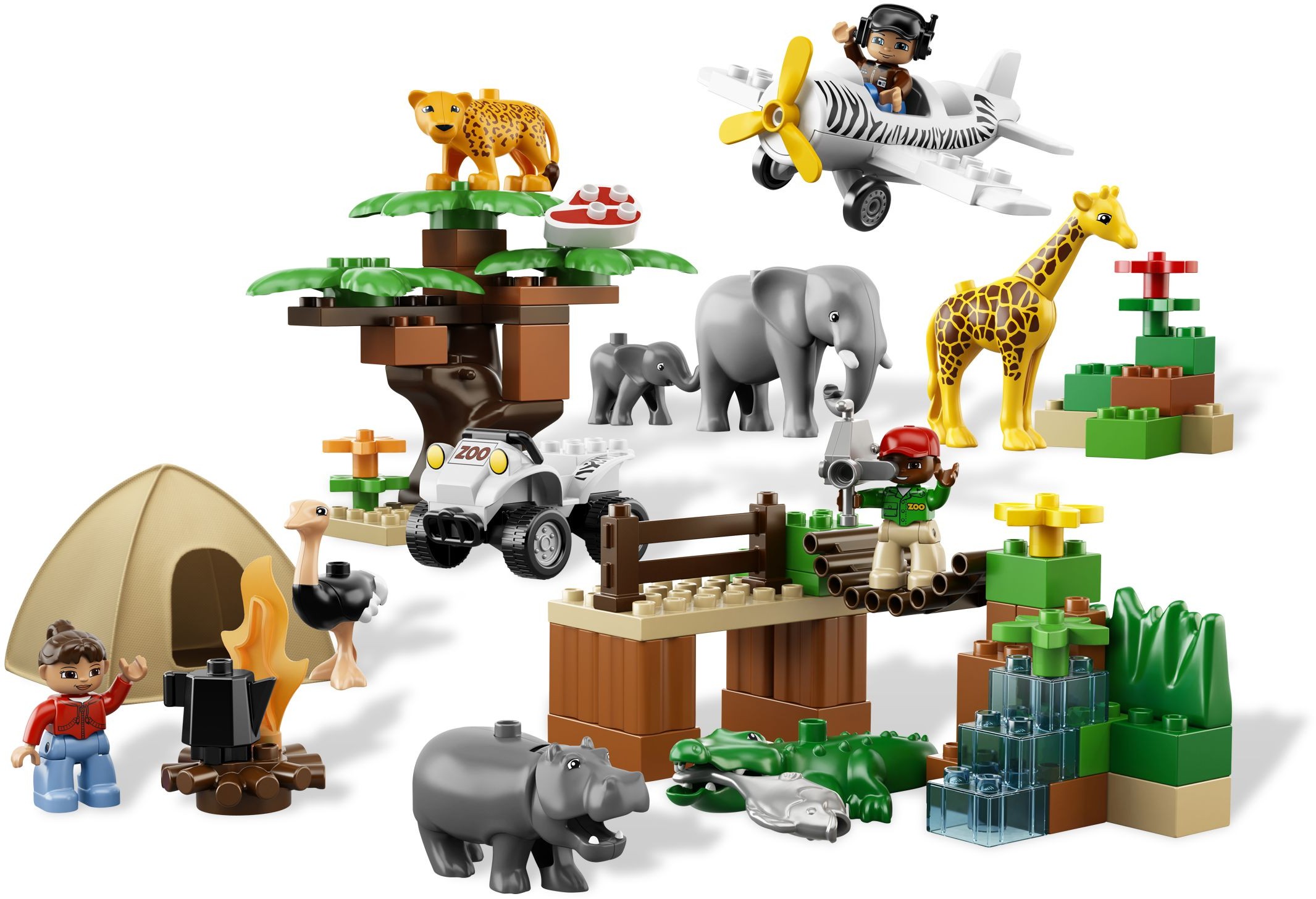The image depicts a vibrant Lego zoo scene set against a white background. At the bottom left, an outdoorsy young girl with brown skin, brown hair, a red top, and blue jeans stands beside a Lego campfire, complete with an orange flame, a brown base functioning as a log, and a black kettle over the fire. Behind her is a tan dome tent, and to its right stands an ostrich with tan skin, black fur, and white feathers.

Moving right, the next grouping includes a zoo truck parked next to a series of Lego trees and bushes. Atop this greenery stands a yellow and black-spotted leopard, although one caption posits it might be a cheetah. Beside these structures are two elephants, a larger one and a baby elephant. 

Above them, a young boy flies a zebra-striped airplane with yellow propellers, wearing a brown helmet or cap. Below the airplane is a yellow giraffe with brown spots.

Further right, a man with black skin, wearing a red cap, a green top, and white pants, peers through binoculars while standing on a bridge above an alligator, which is holding a fish in its mouth. This bridge connects green, red, brown, and light blue structural blocks. The base of the bridge is supported by brown and tan blocks, representing a moat-style structure, enhancing the zoo-like aesthetic.

The entire scene is rich in detail, showcasing a diverse collection of animals, from a tiger or leopard, giraffe, and elephants, to an ostrich and an alligator, amidst a playful, safari-themed Lego landscape full of colorful characters and imaginative setups.